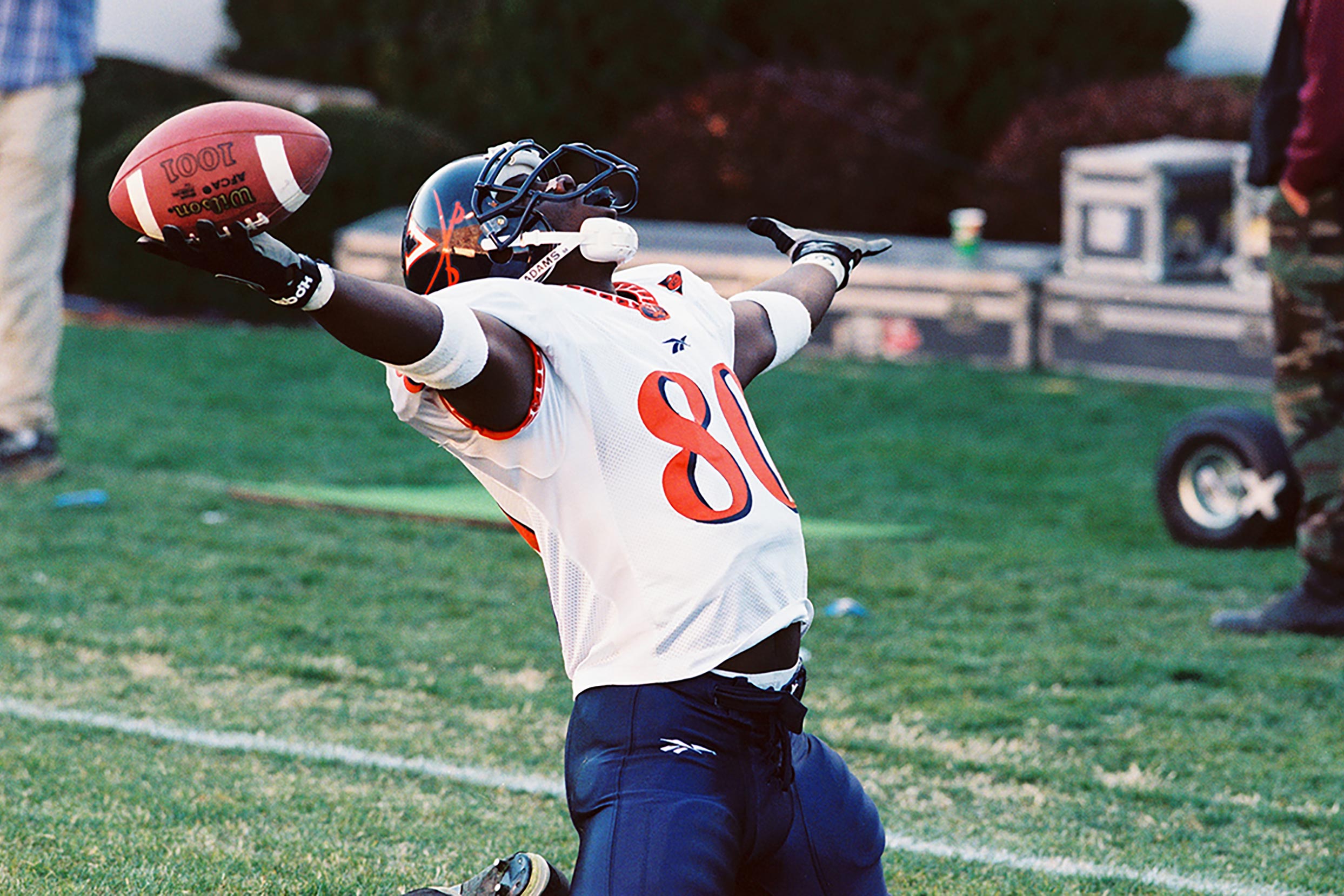A vibrant color photograph captures a dark-skinned football player kneeling on a patchy grassy field. The athlete, donning a white jersey with the bold orange number 80, pairs it with blue tights and white elbow pads. Completing his gear, he sports black gloves, a black helmet with a black face mask, and a white chin strap. He looks upwards, stretching his arms out to both sides in a celebratory pose, clutching the football firmly in his right hand. Behind him, the scene is set with metal chests and two men standing off to the left and right sides. The photo's soft cyan hue and the slightly blurred greenery evoke a sense of dynamic action, possibly hinting at a photograph from a sports magazine.